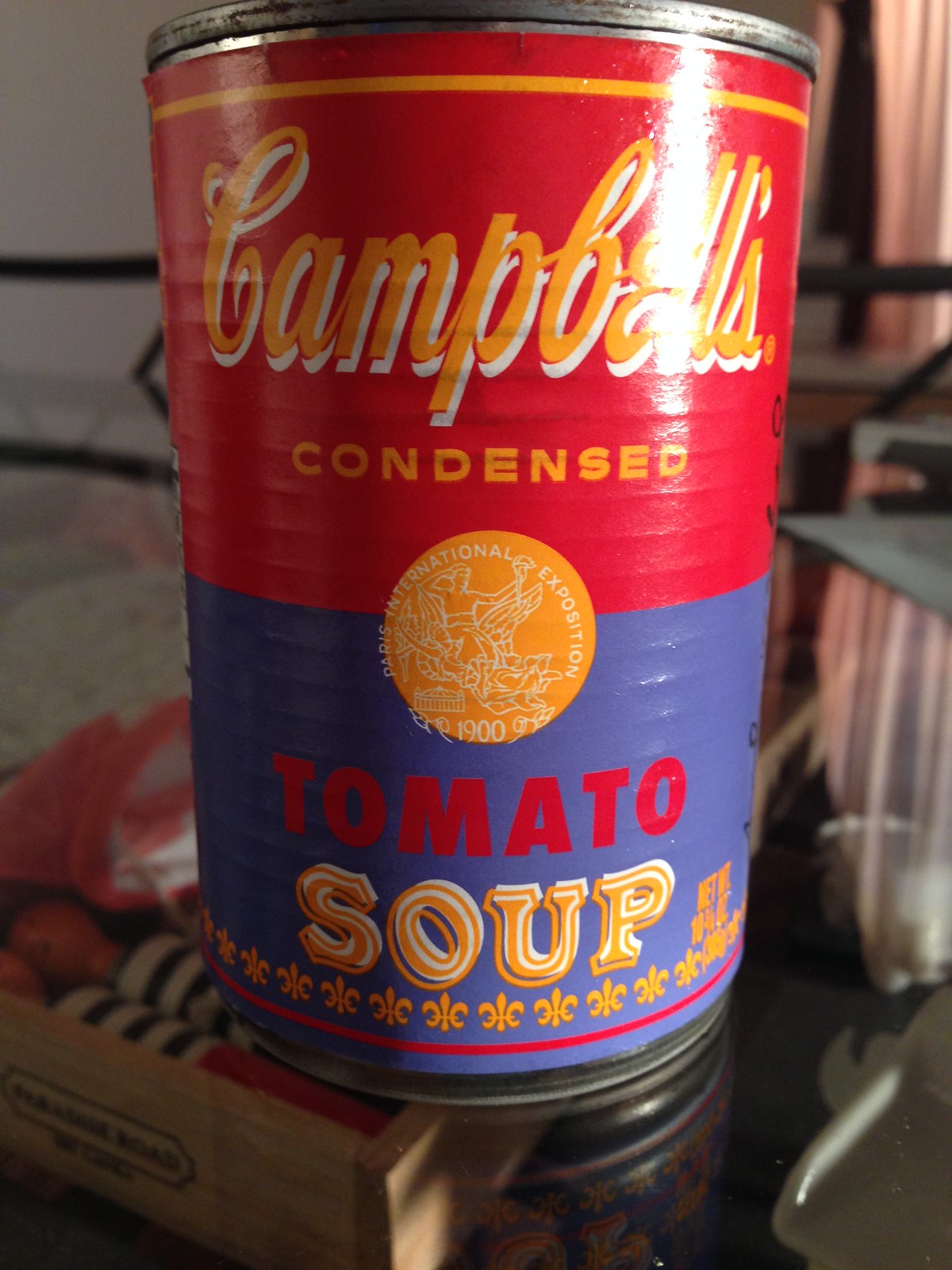This colour photograph, taken indoors in portrait orientation, showcases a close-up view of an aged Campbell's condensed tomato soup can. The can’s metallic top is slightly cut off, with visible rust indicating its old age. The label on the can features a vivid red upper half and a bluish-purple lower half, separated by a yellow strip running horizontally around the entire circumference. 

The iconic Campbell's branding is presented in a stylized manner, with the brand name "Campbell's" rendered in a yellow font that is shadowed by white, giving it a layered effect. Below the brand name, the word "condensed" is displayed prominently. Additionally, there is a seal in the middle, resembling an orange circle with white etching, adding to the vintage feel of the label.

The lower part of the can reads "tomato" in red text and "soup" in a gold-white combination. Surrounding the bottom of the label are several stylized fleur-de-lis designs, contributing to the classic aesthetic of the can. This Campbell's soup can is shown resting on a glass table, further accentuating its nostalgic and time-worn appearance.